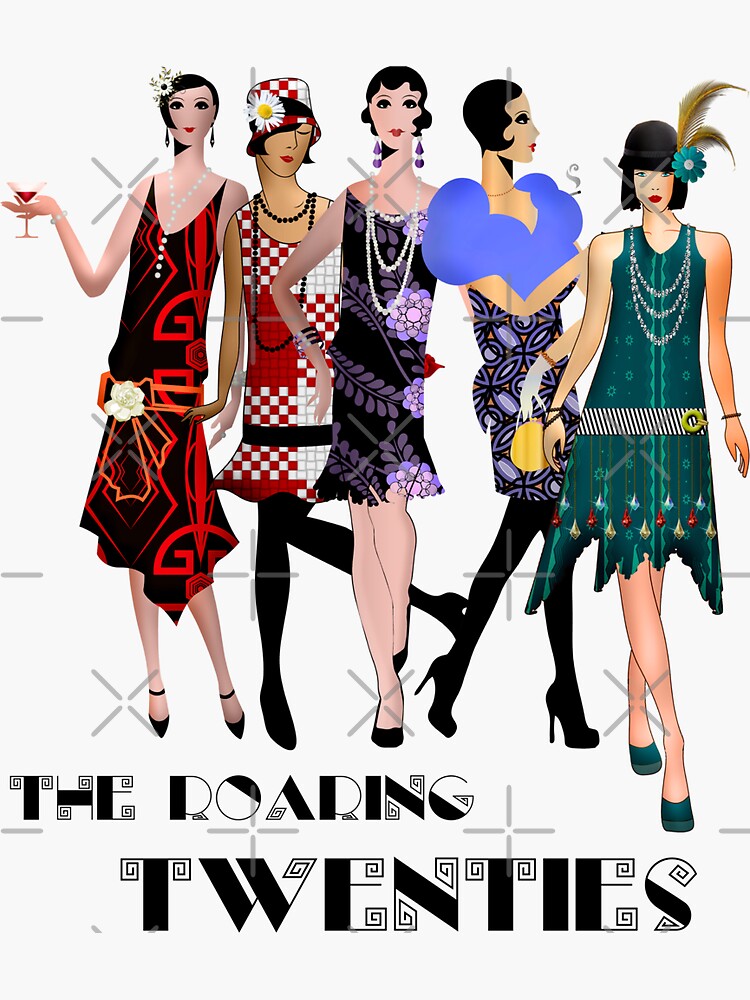The image features a vibrant drawing of five distinct women, all styled as flappers from the Roaring Twenties and set against a white background with light gray marks. Each woman is adorned in unique and colorful attire, showcasing a range of fashion from that iconic era. 

On the left, the first woman holds a martini glass filled with a red liquid in her right hand. She wears a red dress with black accents, a flower at the waist, a matching flower in her hair, earrings, and black shoes. Next to her, the second woman flaunts a red and white checkerboard dress paired with a matching hat adorned with a white flower and yellow center. She completes her look with black socks and black high heels.

The center figure is dressed in a black dress adorned with purple floral patterns and wears black shoes. To her right, another woman sports a black dress with a purplish-orange design, black leggings, and black high heels. Lastly, the woman on the far right brings a pop of color with her green dress featuring white, red, and gold embellishments and a black and white striped belt with a green buckle. She accessorizes with a black hat, silver necklaces, and green high-heeled shoes.

Beneath the elegantly depicted women, a bold and fanciful script reads "The Roaring Twenties," grounding the image firmly in its historical context.